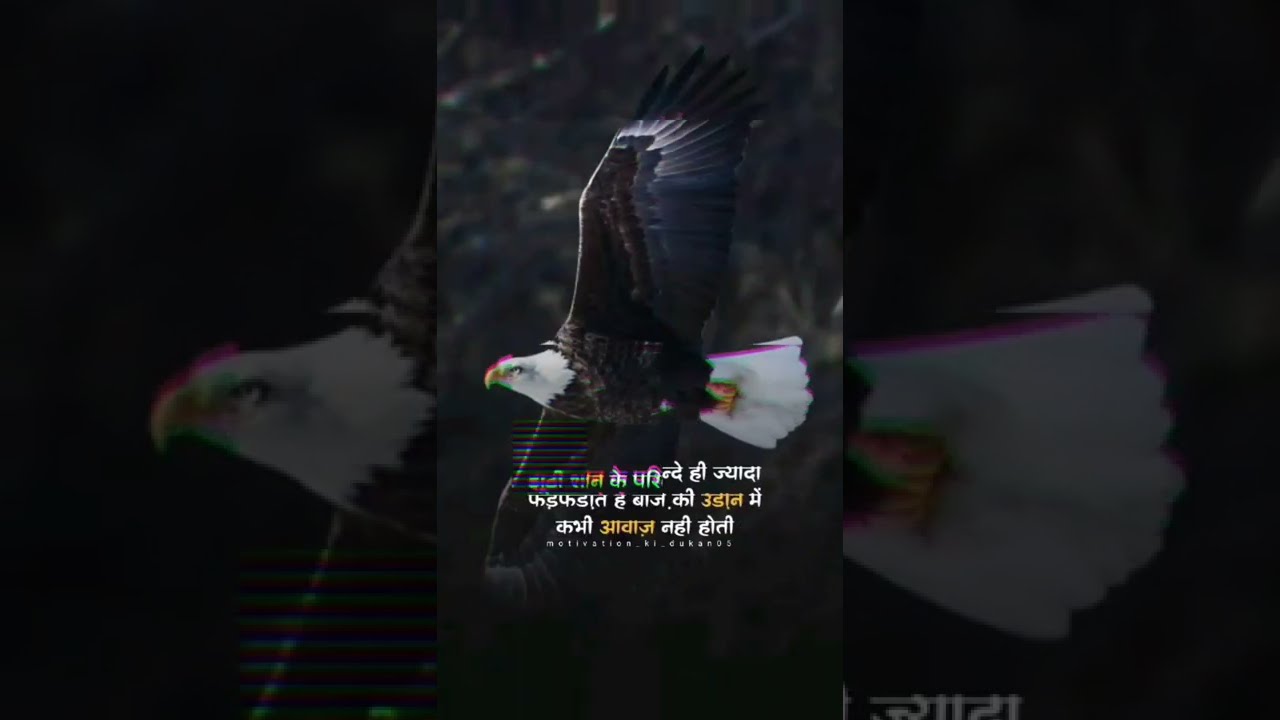A stunning image captures a majestic bald eagle in mid-flight, showcasing the iconic white head and yellow beak of the bird. With its powerful wings fully spread, the eagle reveals its dark brown feathers that contrast with the white feathers at its tail. Its sharp, pointy beak curves downward slightly, and its orange feet are visible against the backdrop of its dark body. The bird occupies a significant portion of the portrait-mode frame, flying from left to right, and set dramatically against a slightly blurred background that hints at a natural environment with indistinct trees. Overlaying the image is a text in an unfamiliar, possibly Indian or Middle Eastern script, featuring both white and yellow characters, with additional smaller text beneath. The overall composition highlights the dynamic movement and grandeur of the eagle, making it the focal point amidst the subtle backdrop.